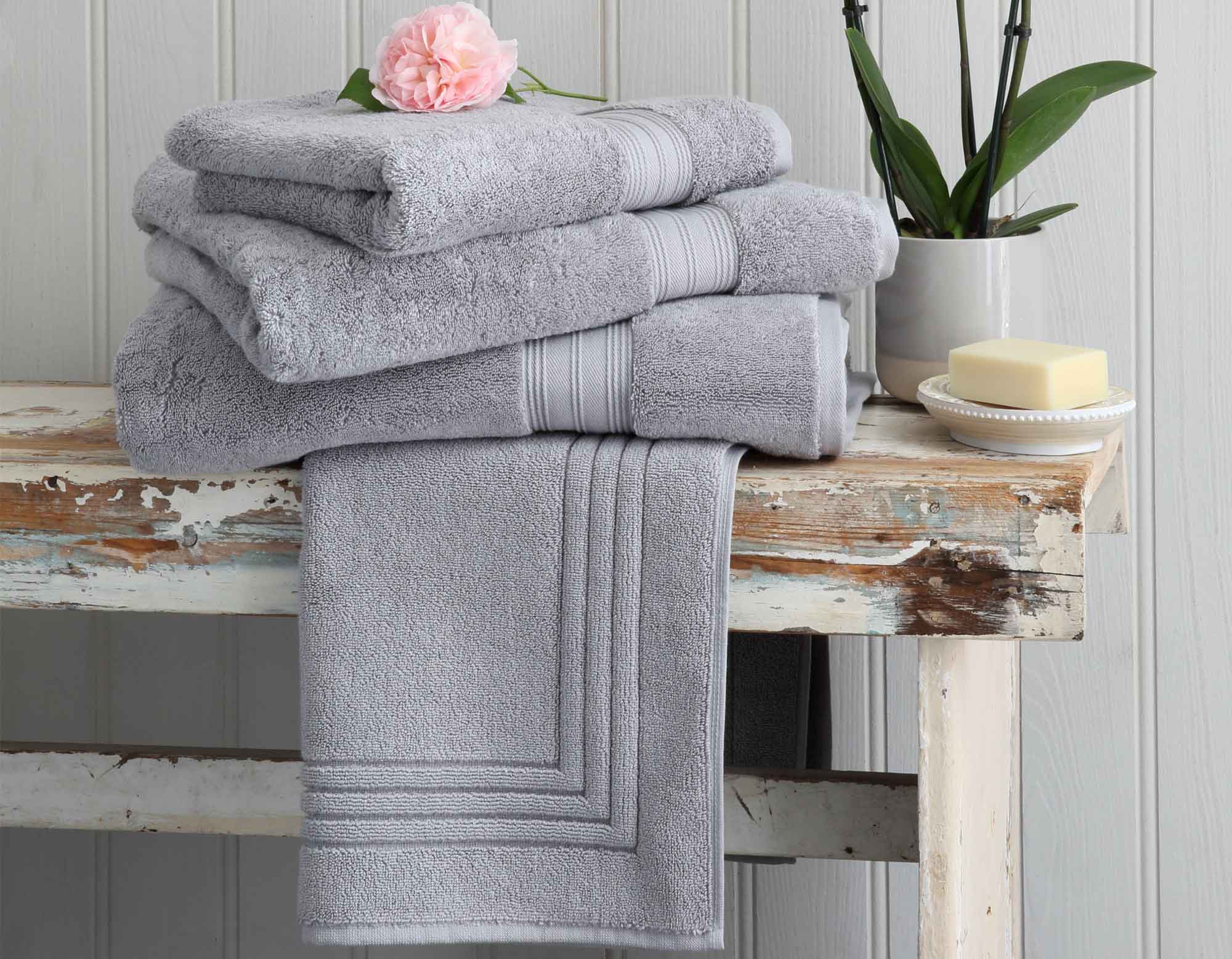The image features a beautifully staged scene with a rustic, shabby chic table made from weathered, reclaimed wood. Once painted white, much of the paint has chipped away, revealing a distressed wood finish. The background showcases white beadboard paneling, adding to the rustic charm.

On the table, a plush gray bath mat hangs down the side. Neatly stacked in the center are three gray bath towels, with a pink carnation adorning the top of the stack. To the right of the towels, there is an elegant white soap dish carrying a bar of cream-colored soap, oval in shape, contrasting with the rectangular soap.

Adding a touch of nature, a small round pot, similar in color to the towels, sits behind the soap dish. It holds a vibrant green plant, possibly an iris or bamboo, with tall stems and broad leaves, extending upwards but remaining out of frame.

The whole composition exudes elegance and is evocative of a high-end catalog display for bath linens.